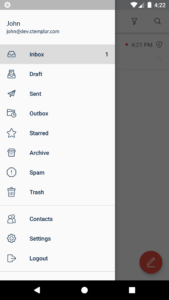The image depicts a mobile email application interface. At the very top, there is a gray navigation bar, which includes indicators for Wi-Fi signal strength and battery level, both showing full status, along with the current time displayed as 4:22 PM. The upper-right corner also features an icon set typically found on smartphones. 

Directly beneath the gray bar on the left side, there’s a wider white strip featuring the name "John" and an email address that starts with "John" followed by "at" and an obscured domain due to poor resolution, making it unreadable. 

The main portion of the screen shows a vertical menu on the left side of the display, with options like Inbox, Drafts, Sent, Outbox, Starred, Archives, Spam, Trash, Contacts, Settings, and Log Out. Each menu item is left-justified, with "Inbox" being highlighted by a gray bar while the background remains white. The Inbox also has a numerical indicator showing the number "1," suggesting there is one unread email.

On the bottom right corner of the screen, there is a red circular icon with a pencil, indicating the option to compose a new email. There are also icons representing a funnel, likely for filter options, and a magnifying glass for searching. 

Lastly, at the very bottom, there’s a black line, possibly part of the phone's physical design or another navigation element of the app interface.